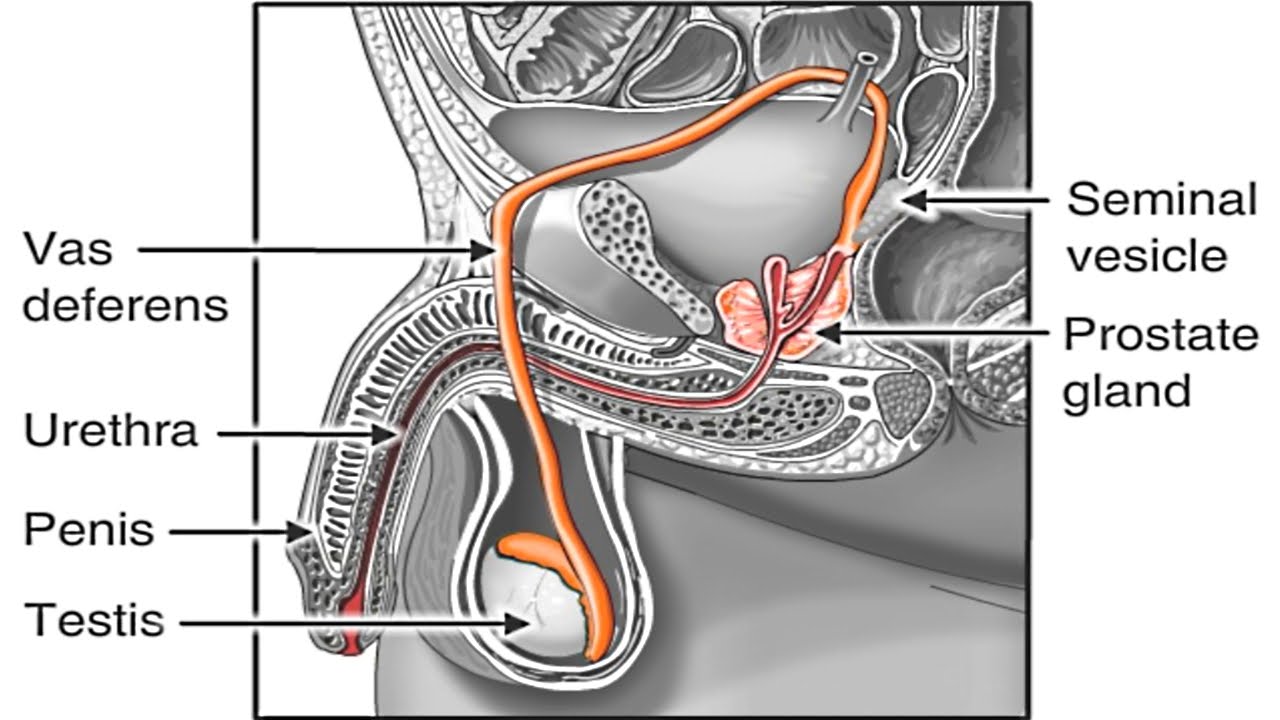This is a detailed, computer-generated, black-and-white medical diagram of male genitalia, presented in a square format with a white background. The illustration, which takes the form of a cross-section, labels several key anatomical structures using arrows. The labels include the vas deferens, urethra, penis, testes, seminal vesicle, and prostate gland. The areas labeled as the seminal vesicle, prostate gland, urethra, testis, and inside of the penis are highlighted in orange, light pink, red, white, and red, respectively. Additional anatomical details such as the bladder, bone, and skin are also depicted, with some parts labeled in a language other than English. This diagram resembles those typically found in encyclopedias, dictionaries, or science textbooks, providing a comprehensive view of the male reproductive system.